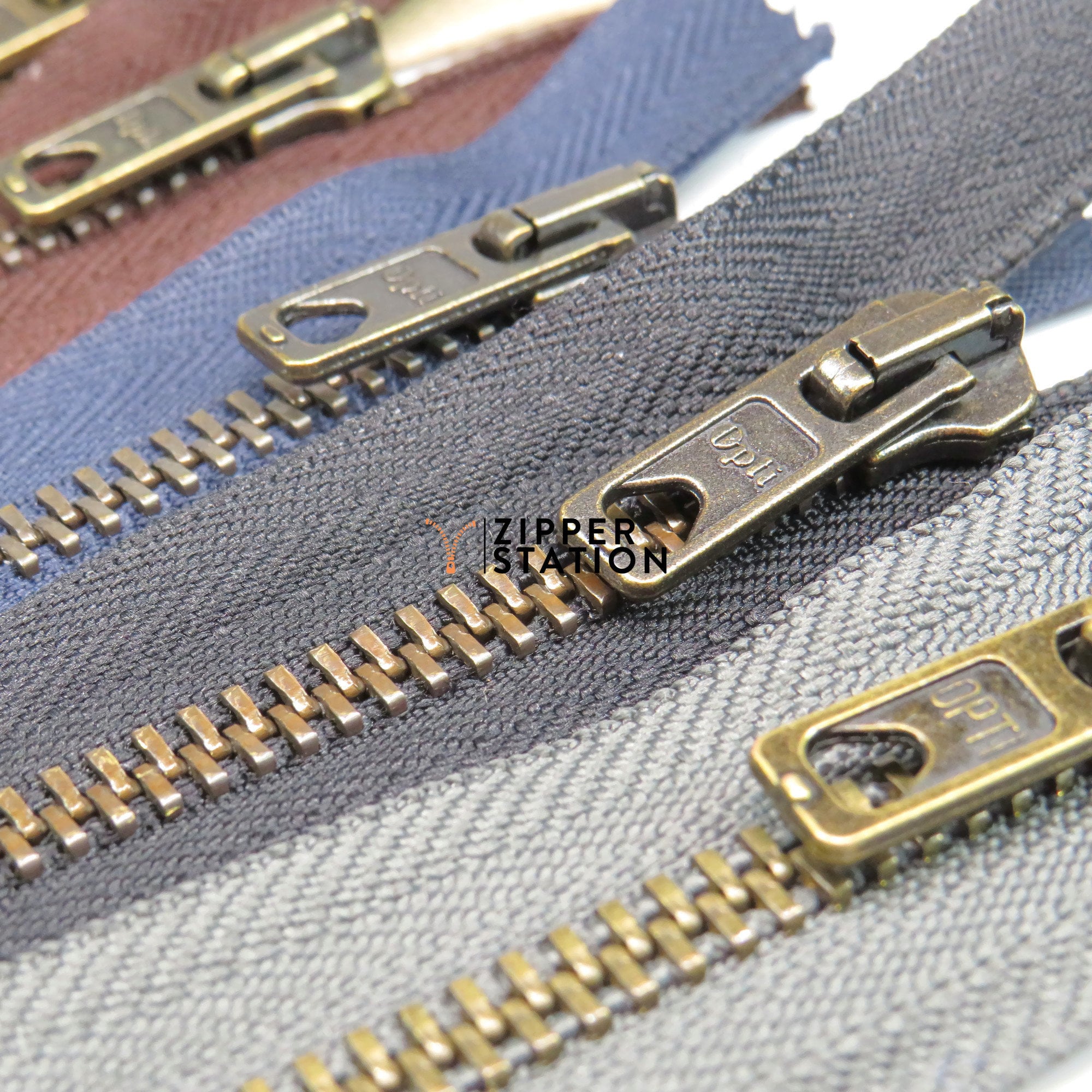This image is a close-up photograph of five zippers, each in a brownish-bronze or brass color. The zippers are arranged from the top right corner to the bottom left, with their handles above the closed teeth. Each zipper is attached to a different colored fabric: the bottom right one is light gray, followed by a darker gray fabric, then a light blue fabric, and finally, a burgundy or light maroon fabric. The fabrics and zippers are arrayed on what appears to be a white table, visible in the upper right corner. The zipper tabs bear the brand name "OPTI." Overlaying the image, there's black text reading "Zipper Station" in two lines, with a thin black vertical line beside it. To the left of the text is a small, orange cartoon depiction of a zipper forming a V-shape as it is being pulled open.